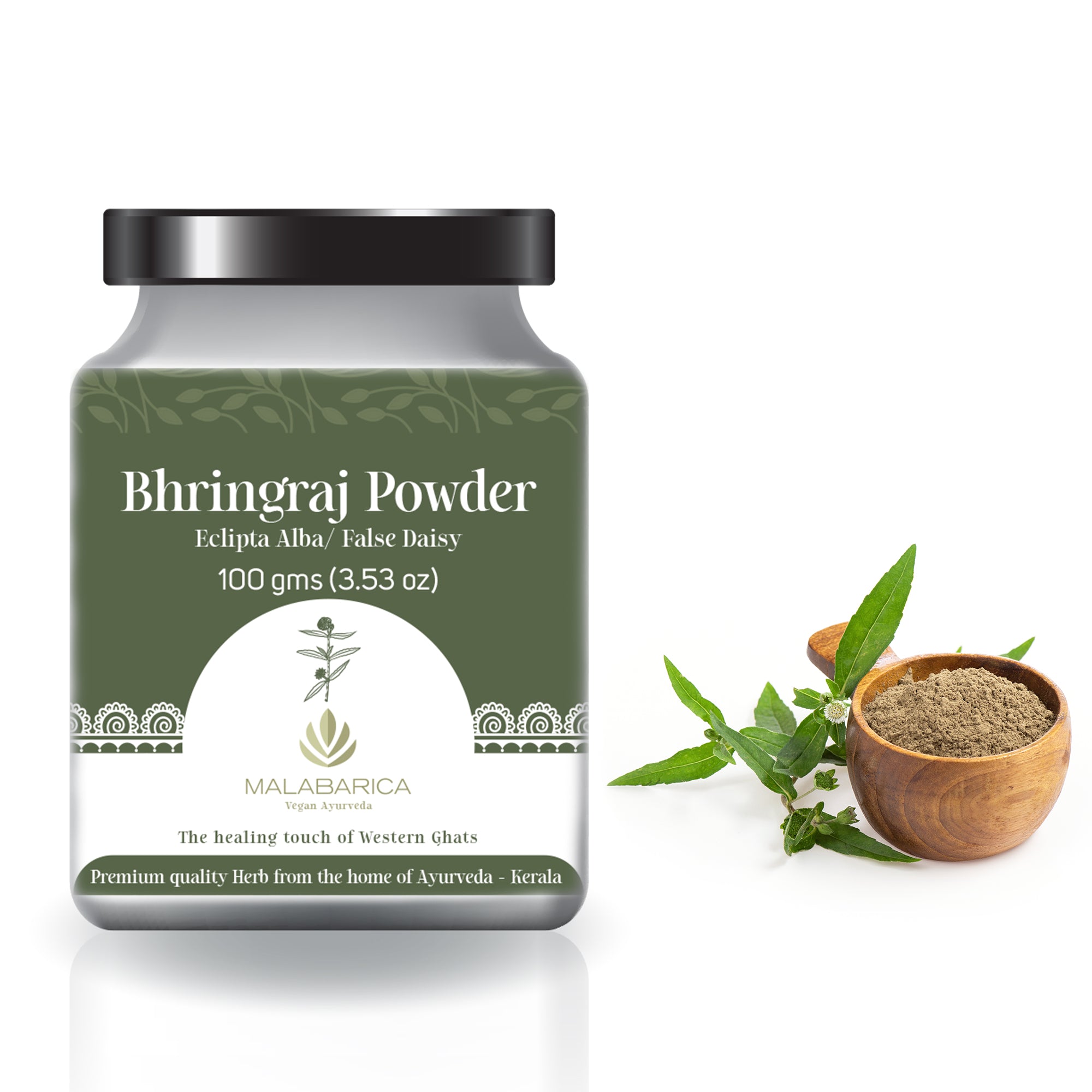The image features a bottle on the left side and a wooden bowl filled with finely ground brown powder on the right. The wooden bowl is round with distinct circular lines along its sides. Next to the bowl is a green leafy plant. The bottle, positioned far to the left, has a square-shaped body with a black cap. It has a green background and reads "Bhringraj Powder, Eclipta Alba / False Daisy, 100 gms, 3.53 oz." Below this, there's a white circle with a flower inside it, accompanied by green stems and leaves. Further text on the bottle includes "Malabarica" and "The Healing Touch of Western Ghats," followed by "Premium quality herb from the home of Ayurveda, Kerala" at the bottom. The bottle is primarily gray with a green band around the middle featuring plant leaves. The photograph appears to have been taken looking directly at these items against a plain, likely digitally created white background. The powder in the bowl is notably fine, and the photo of the plant and bowl is taken from above at an angle. The color palette includes dark green, light green, white, black, light brown, and tan.